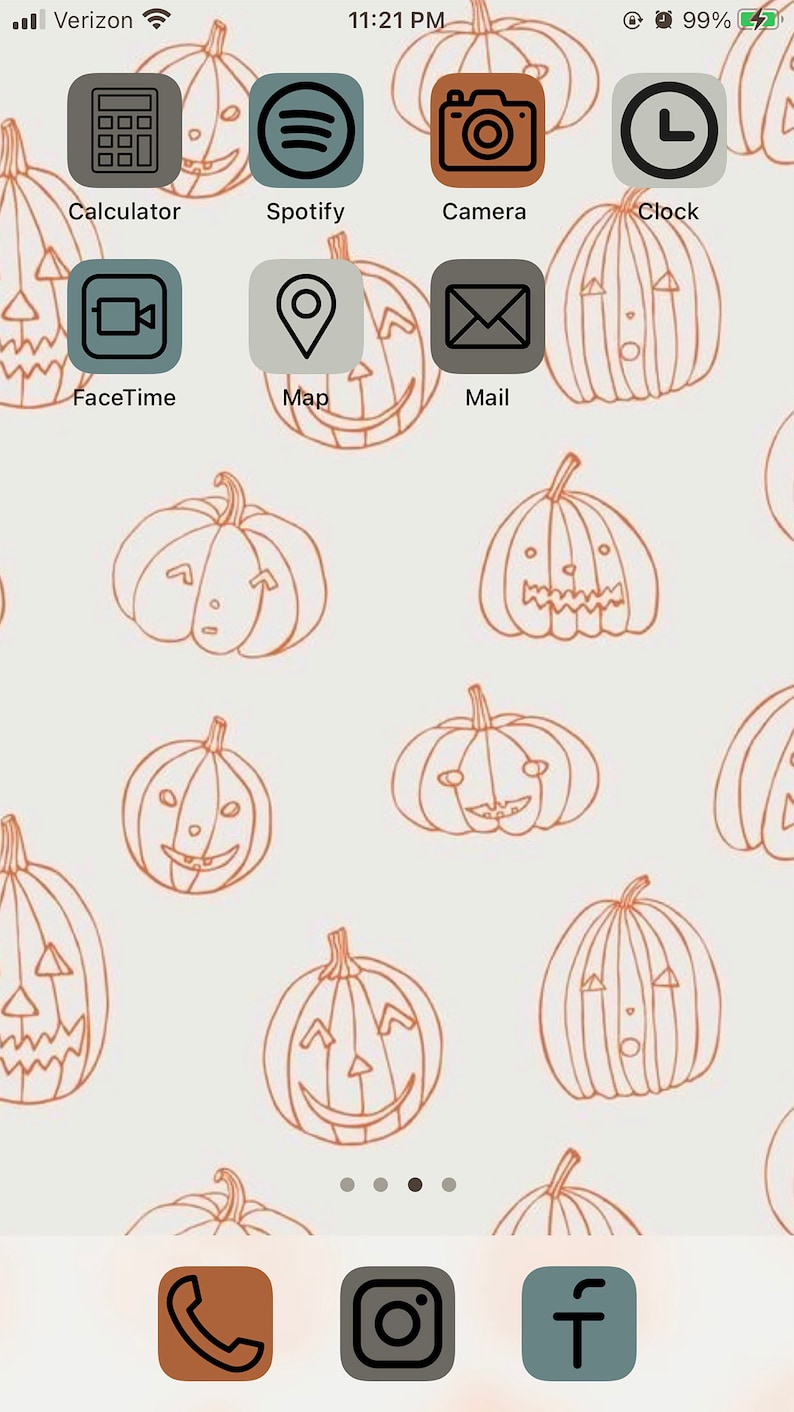This image captures an Apple iPhone home screen featuring a delightful fall-themed background. At the very top, the status bar displays the cellular signal on the left, indicating Verizon as the carrier, with the Wi-Fi symbol on the right. Centered in the status bar, the time reads 11:21 p.m., and the battery icon shows 99% and charging, alongside an alarm icon.

The home screen background boasts a light gray or beige hue adorned with orange jack-o'-lanterns, each sporting various expressions ranging from spooky to faintly smiling to blank. This seasonal theme extends to the app icons, which are colored in shades of gray and orange to match the fall aesthetic.

Prominently arranged icons on the screen include those for Calculator, Spotify, Camera, Clock, FaceTime, Maps, and Mail. At the bottom of the screen, the dock features the Phone, Instagram, and Facebook apps. This detailed autumn scene combines practical information with festive, whimsical design elements, creating a visually appealing and functional interface.